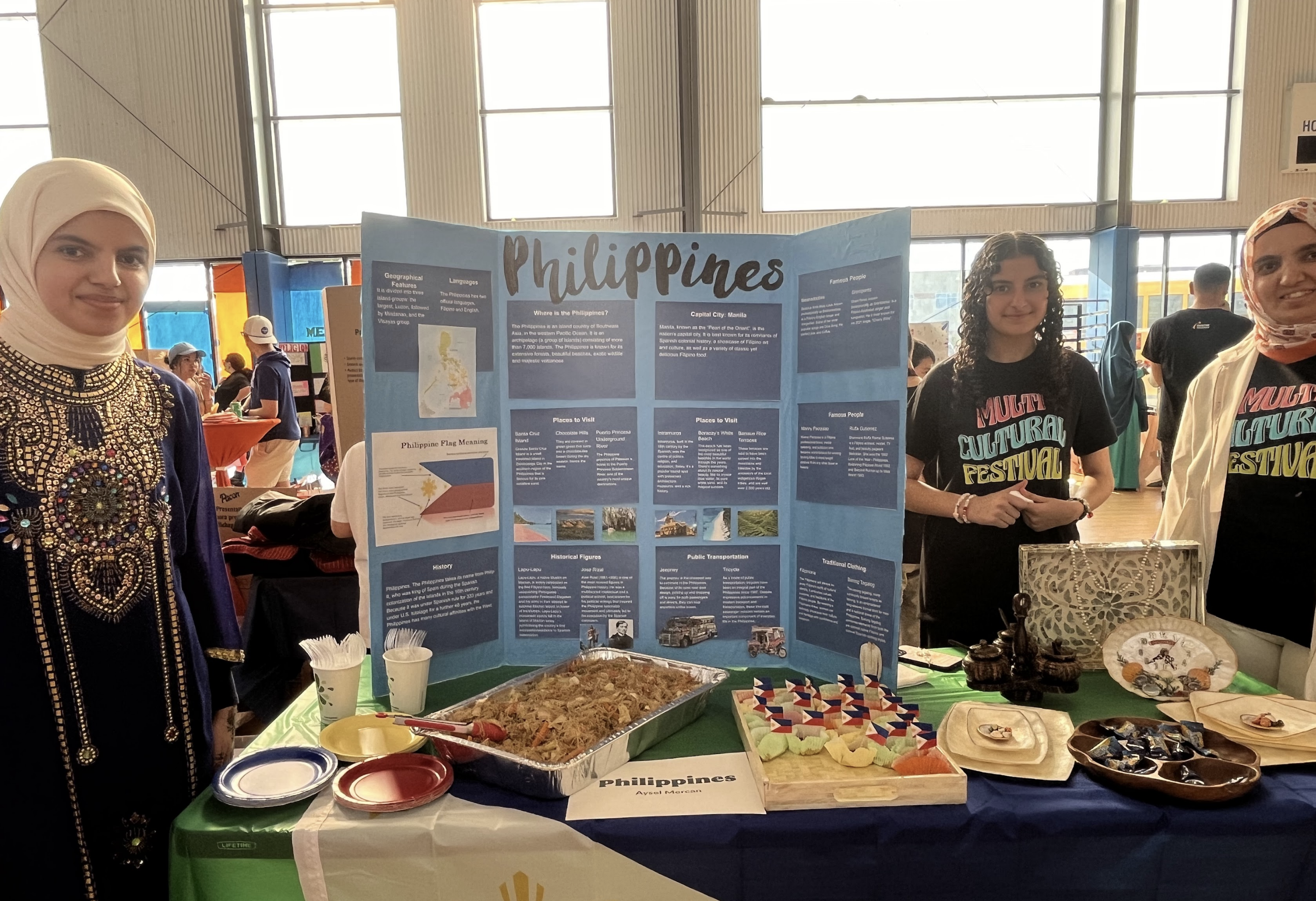The image depicts a vibrant scene at a multicultural festival, focusing on three young female students presenting an exhibition of Filipino cuisine. The central part of the scene is dominated by a large, folded cardboard display board titled "Philippines" in black letters. This trifold is covered with diagrams, text, and an image of the Philippine flag, though the smaller details are not legible. The table in front of them is adorned with various trays of Filipino food, including noodles and beef in a rectangular foil tray and a wooden tray with small flags sticking out of the food items. The table also has colorful paper plates in blue, red, and yellow, along with plastic utensils for attendees to use.

Two of the young women are wearing black t-shirts emblazoned with "Multicultural Festival" in pink, blue, and yellow letters. One of these women is on the right side of the image, wearing a scarf over her head. The third woman, on the left, has brown hair, is smiling at the camera, and is dressed in a dark blue gown decorated with intricate beading, complemented by an ivory-colored scarf wrapped around her head and neck.

In the background, there are other tables with similar trifold displays and more students, adding to the festive and educational atmosphere. The backdrop includes large windows through which a cloudy sky and part of a bus are visible. Additionally, an array of colors such as blue, black, white, red, green, yellow, and peach, along with gold emblems on a purple and white banner, enriches the visual complexity of the scene.